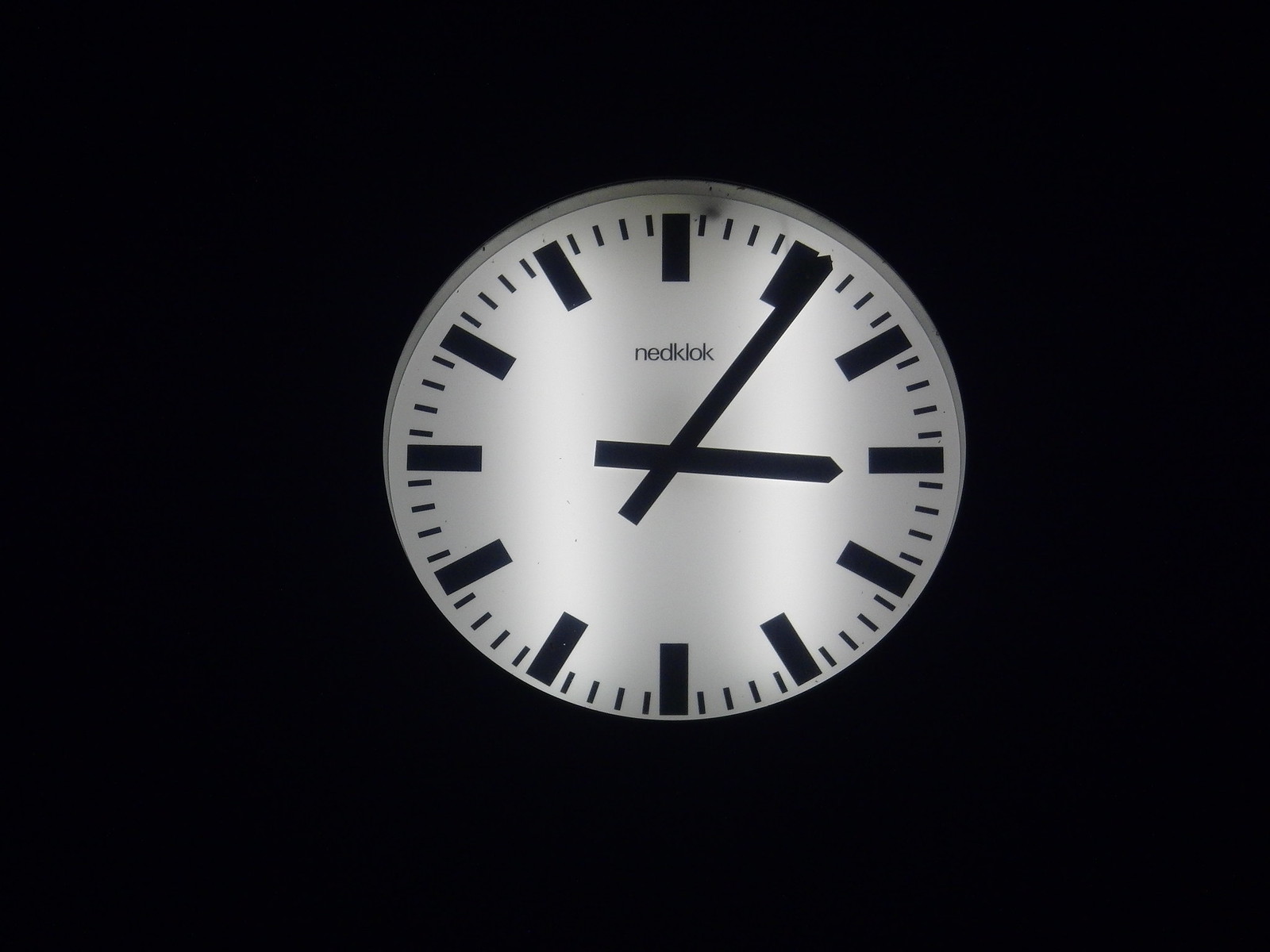In this image, we observe a minimalist clock design set against a solid black background, emphasizing the clock as the striking centerpiece. Encircling the clock face, instead of traditional hour numbers, there are sleek, rectangular black markers denoting each hour from 1 through 12. Positioned just beneath the 12 o'clock mark is the brand name "NEDCLOCK," spelled N-E-D-C-L-O-K. The clock hands are centrally aligned, with the short hour hand pointing at the 3 o'clock position and the longer minute hand directed at the 1 o'clock position. Between each of the rectangular hour markers, there are four dashed lines indicating 15-minute increments, enhancing the clock's precision and design clarity. The entire scene is framed by a solid gray line tracing the periphery of the clock face, creating a subtle contrast against the black background.